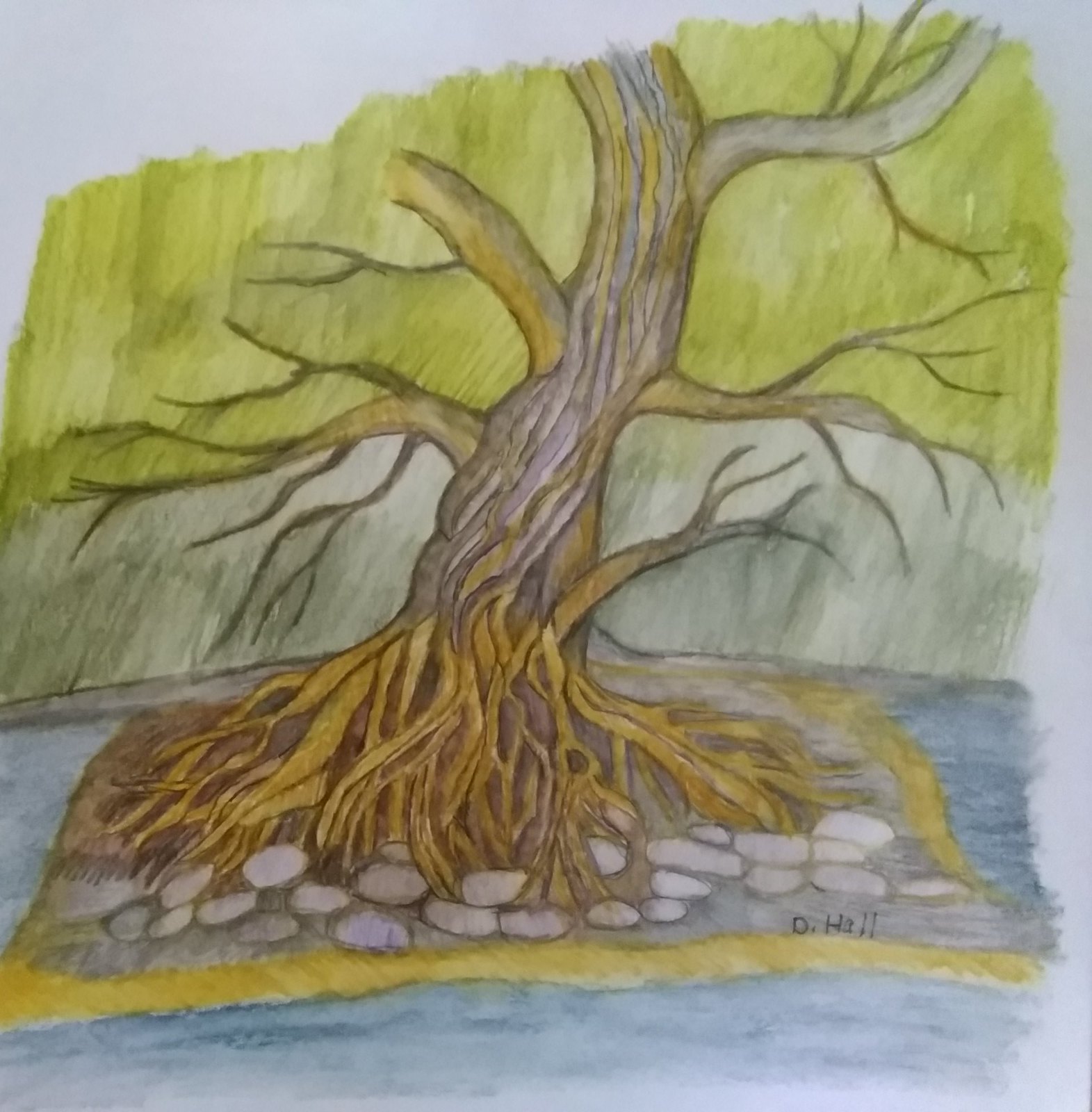In the center of the illustration stands a prominent tree with dark brown bark and sprawling roots, tinged in a yellow hue, extending downward. Surrounding the tree is a body of water, rendered in a rich blue shade. Encircling the water is a yellow border, resembling dirt, which is then surrounded by an array of meticulously drawn stones. At the bottom right of the image, Dr. Hall is depicted, adding a human element to the scene. The tree's branches extend outward with green leaves at the top, contrasting with the dark shadowing at the midsection and the white highlights on the uppermost branches. The entire composition appears to be created using markers or similar coloring tools, giving the artwork a vibrant and textured appearance.